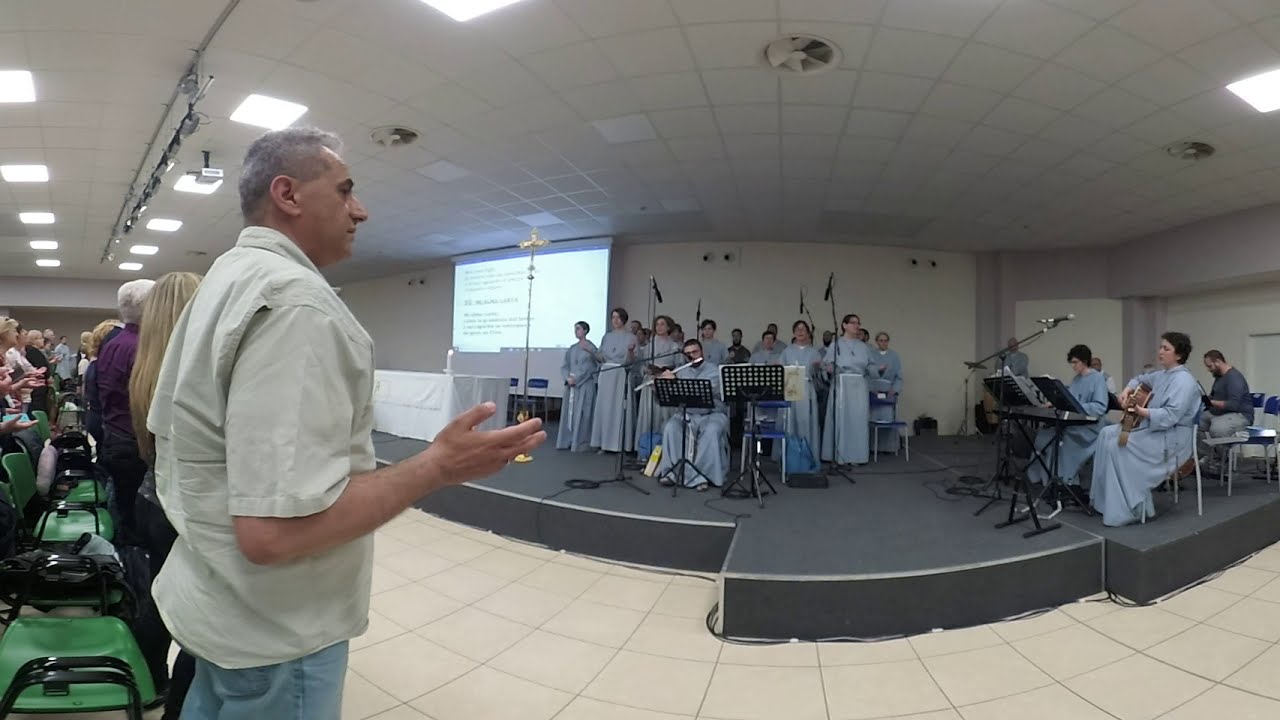This detailed, photographic image captures a vibrant church service taken with a wide-angle lens, giving the scene a slight curvature. In the foreground, on the left-hand side, a man with white hair, wearing a short-sleeved shirt and blue pants, stands with his arms raised and palms upward, echoing the posture of the other congregants around him. Behind him, a blonde woman and another white-haired man are also visible, immersed in the service. The congregation, predominantly composed of elderly women with white hair, all have their palms raised towards the ceiling, which features a dropped design with recessed fluorescent lighting.

The focal point of the image is a gray-carpeted, silver-trimmed stage. Here, a chorus of men and women stand in two rows, all donned in blue robes with white sashes. At the center of the stage, a man seated with a flute plays energetically, while other members of the group sing with some holding microphones or music stands. To the right of the chorus, several individuals are engaged with musical instruments—a woman strums a guitar, another plays the keyboard, and a man in a gray sweatshirt and pants, who is not robed, may also be participating despite his ambiguity. The latter has a beard and mustache, adding diversity to the ensemble.

In the background, a projection screen displays text that remains unreadable due to its blur. Additionally, to the left of the choir, a white table adorned with a long tablecloth and a candle adds a liturgical element to the setting, enhancing the church-like ambiance. This image profoundly captures the unity and devotion of the participants, centered around music and worship within a warmly lit church environment.